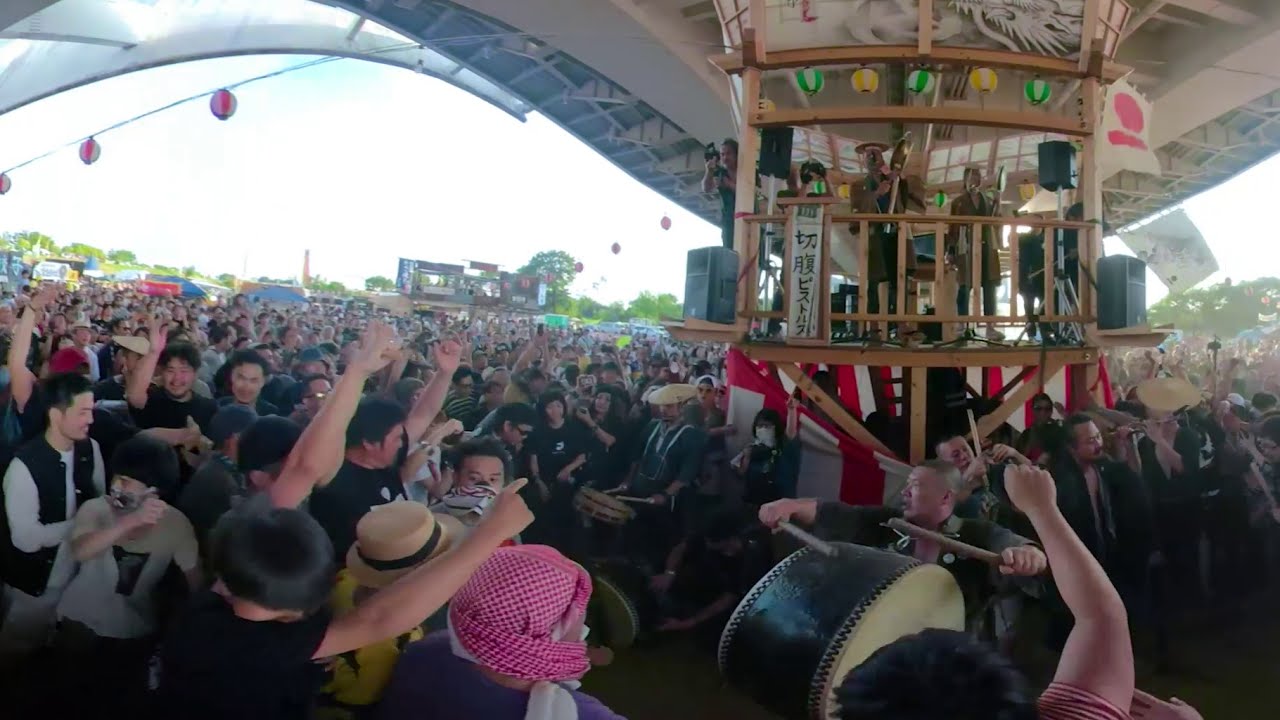Captured in a vibrant outdoor music festival in East Asia, possibly China or Japan, this lively scene features a small, circular wooden stage at its center. This stage, described as a bit makeshift, hosts a group of traditional musicians clad in unique, flat hats reminiscent of dinner plates. The musicians are surrounded by an enthusiastic crowd that numbers in the thousands, their energy palpable as they raise their arms and cheer. The festival's atmosphere is electric, amplified by numerous speakers positioned around the stage and a white banner adorned with Asian characters flying above. The open-air venue offers glimpses of a clear blue sky and lush green trees in the background, while the event appears largely covered by a roofed pavilion without walls. Adding to the festive ambiance are colorful balloons in shades of green, yellow, and pink scattered throughout the scene. In the distance, an infotainment screen and small shops are visible, enhancing the communal, celebratory vibe of this large-scale cultural event.